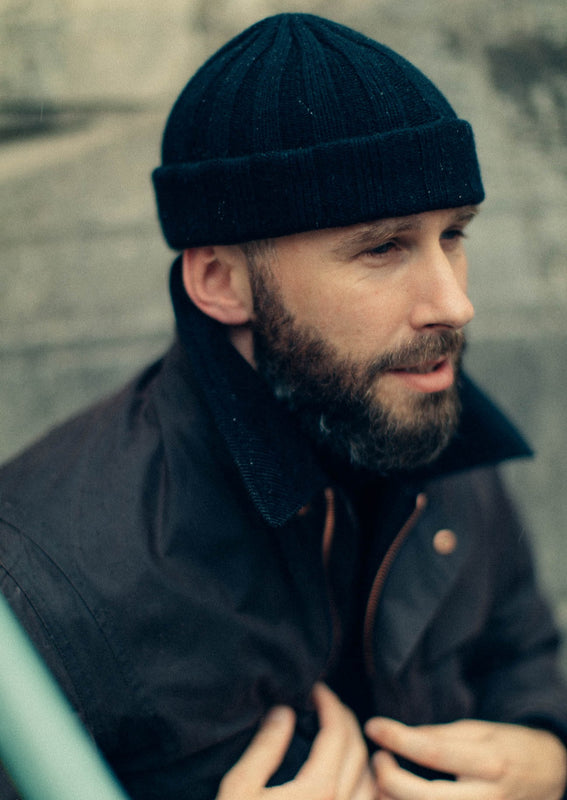This portrait captures a white male with pale skin and brown scruffy facial hair, including a beard and mustache. He is wearing a snug-fitting black beanie that covers most of his ears and reaches down to his eyebrows. His expression is one of distant contemplation, with his eyes squinting slightly as he gazes out towards the right side of the frame.

The man is dressed warmly, implying a cold setting. He dons a dark navy or black jacket, which features a collar and copper or brass buttons. His hands are visible at the bottom of the image, holding the jacket around the center, possibly in the process of zipping or adjusting it. 

The background is a blurry, nondescript gray, making it difficult to discern any specific location details. A light green bar, out of focus and at a 45-degree angle, can be seen at the bottom left of the image, adding a slight contrast to the otherwise muted backdrop.